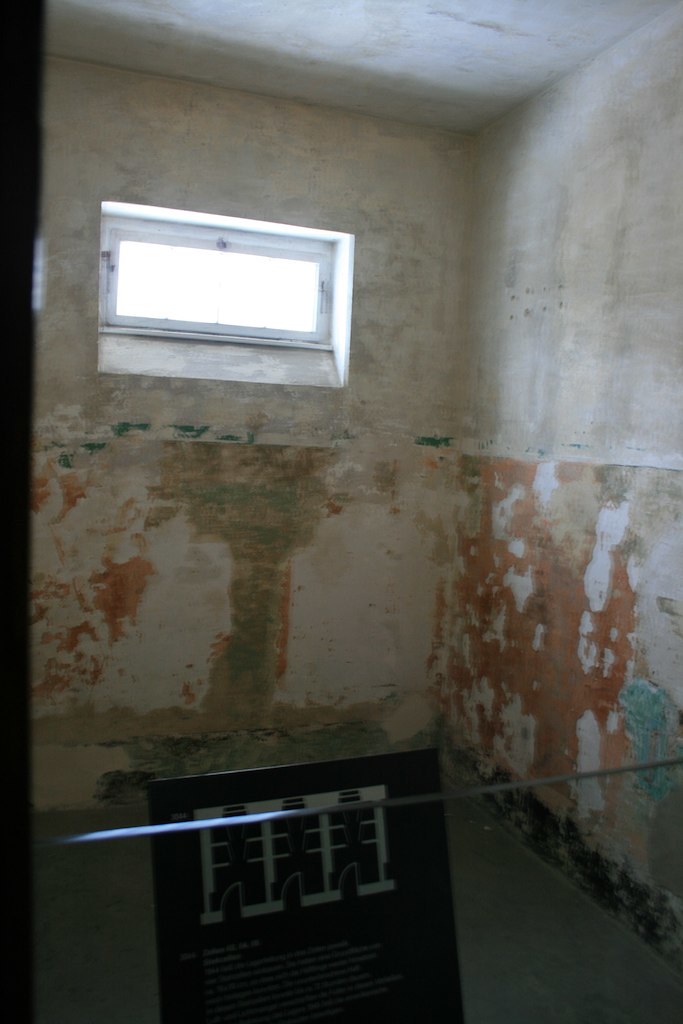The image depicts a worn and aged room with predominantly white plaster and paint, now significantly peeling and marked by brown and green-gray patches indicating considerable decay. The room appears to be part of an old building, possibly an exhibit of a historical site, such as a former prison cell open to visitors. A rectangular window, wider than it is tall, is located at the upper left portion of the room, allowing bright light to seep through, which appears more like fluorescent light than sunlight. The upper half of the room's walls is noticeably cleaner, with a sandy stone color close to gray or light brown, whereas the lower half is heavily chipped and stained, with blotches including an orange water stain. Below the window, a small rod runs horizontally across the image, with a black sign resting on the floor behind it, providing historical information about the room’s past usage. The overall environment is very decrepit, echoing a long history and previous utilitarian function, now maintained as an exhibit for educational or memorial purposes.